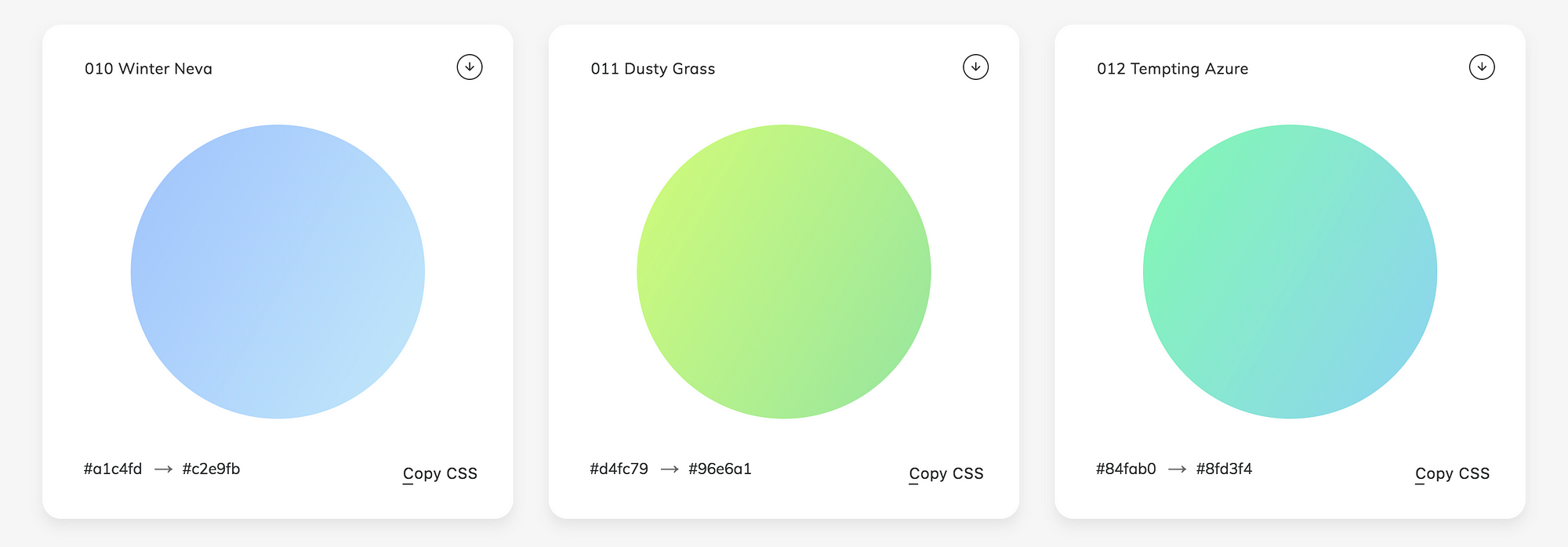This image is organized into three distinct square sections, each featuring unique elements, colors, and identifiers:

1. **Left Square:**
   - **Title:** "010 Winter Nevo" positioned at the top.
   - **Main Feature:** A light blue circle centered in the square.
   - **Annotations:** 
     - Bottom section contains the text "#OLC4FD" followed by a right-pointing arrow, and then "#CDE9TB."
     - "Copy CSS" is located in the bottom right corner.

2. **Center Square:**
   - **Title:** "011 Dusky Gross" located in the upper left corner.
   - **Main Feature:** A green circle.
   - **Annotations:**
     - Bottom section contains the text "#DFD4FC79" followed by a right-pointing arrow, and then "#96E601."
     - "Copy CSS" is placed in the bottom right corner.

3. **Right Square:**
   - **Title:** "012 Tempting Azure" positioned in the upper left corner.
   - **Main Feature:** A circle in a greenish-blue shade.
   - **Annotations:**
     - Lower left corner features the text "#84FABO" followed by a right-pointing arrow, and then "#8FD314."
     - "Copy CSS" is placed in the bottom right corner.

All three squares maintain a consistent layout with color circles at their centers and detailed metadata at the edges, providing a visually structured and informative presentation.